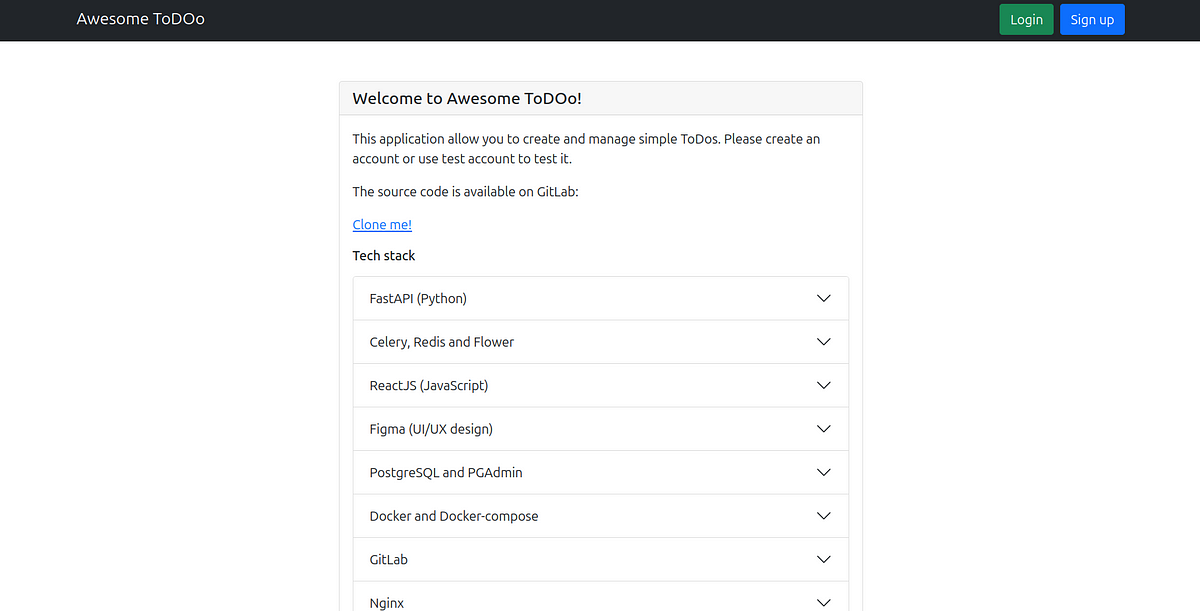The image displays a webpage titled "Awesome To Do," with the title stylized as "Awesome T O Do" (with a capital 'T,' a capital 'D,' and a lowercase 'o'). This title is positioned within a black bar at the top of the page. In the top right corner of the black bar are two buttons: a green button labeled "Log In" and a blue button labeled "Sign Up."

Below the black bar, the page features a white section with additional content. At the top of this section, a prominent heading reads "Welcome to Awesome To Do." Below this, a message explains that the application allows users to create and manage simple to-do lists. It invites users to either create an account or use a test account to explore the features. Additionally, it mentions that the source code for the application is available on GitLab, accompanied by the phrase "Clone me!" which is highlighted in blue and underlined.

Further down, the page lists the technologies used in developing the application, under the heading "Tech Stack." This section displays several boxed items, each containing the name of a technology. The technologies listed include:

- FastAPI (Python)
- Celery
- Redis
- Flower
- React.js (JavaScript)
- Figma (UI/UX design)
- PostgreSQL
- PgAdmin
- Docker
- Docker Compose
- GitLab
- Nginx